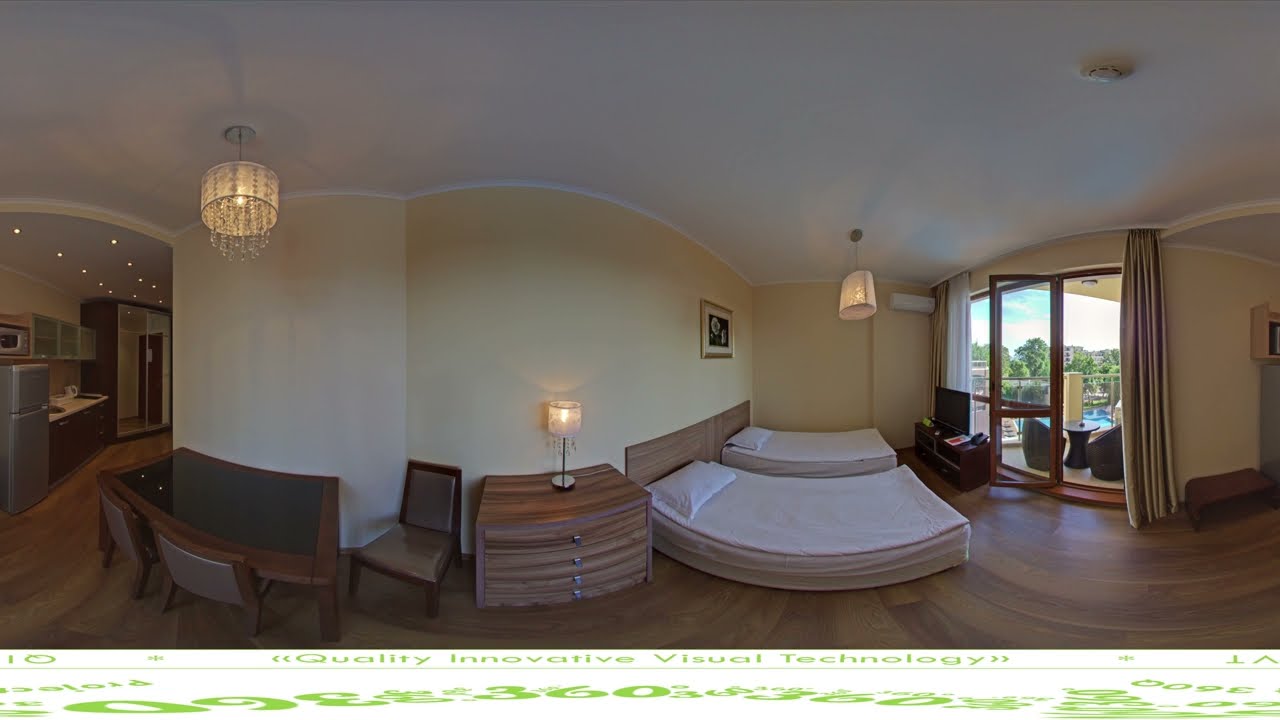This outdoor photograph captures a serene pool deck at a large, resort-style hotel under a crystal-clear blue sky. The image showcases a vivid scene, enhanced with stitching effects that seamlessly merge parts of the photo, particularly noticeable where two sun umbrellas meet in the center top. A distinctive white border frames the picture, with green print at the top reading, "quality innovative visual technology." Along the bottom border, the number "360" appears twice in green print, with an additional inverted "360" on the left.

Underneath the umbrellas providing shade, a tranquil pool lies ahead, its still, blue waters inviting and empty of people. Surrounding the pool is a tiled deck featuring long, light-brown lounge chairs accompanied by matching brown tables with glass tops. The hotel's architecture, standing tall and wide with numerous windows, is highlighted in a mix of yellow and brown hues. Lush grassy areas and trees frame the pool, enhancing its resort-like ambiance. The day is bright and clear, further emphasizing the crystal blue water of the pool and the picturesque setting.